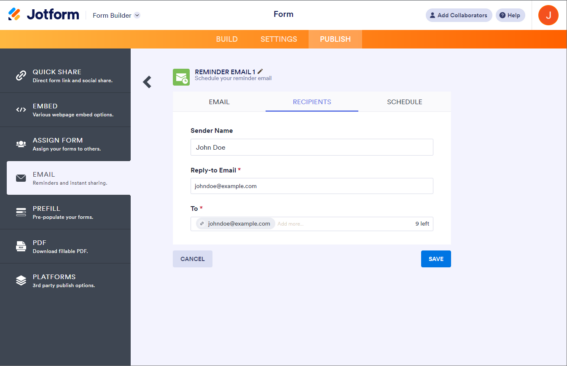The image depicts the interface of JotForm's form builder application. In the top left corner, the JotForm logo featuring a pencil icon in green, orange, and yellow is displayed next to the name "JotForm" written in blue. Centrally positioned on the page, the header reads "Form."

In the top right corner, there are two buttons: "Add Collaborators" and "Help," followed by a profile icon with an orange background and the initial "J" in the center. Below these, there is a yellow toolbar featuring three buttons: "Build," "Settings," and "Publish," with "Publish" being highlighted.

On the left side of the interface, a navigation menu is open, displaying several options:
1. "Quick Share" for direct form links and social sharing.
2. "Embed" for various webpage embedding options.
3. "Assign Form" to delegate the form to others.
4. "Email" for sending reminders and instant sharing.
5. "Prefill" for population pre-forms.
6. "PDF" for downloading writable PDFs.
7. "Platforms" for third-party publishing options.

In the center, the "Email" section is open, titled "Reminder Email 1." It provides options to schedule a reminder email with buttons for "Email Schedule" and "Recipient." In this particular instance, the recipient is selected. The form includes fields such as "Sender Name: John Doe" and "Reply-to Email: johndoe@example.com," along with a field to select the recipient email.

At the bottom right, there are two buttons: "Cancel" on the left and "Save" on the right, with the "Save" button highlighted in blue.